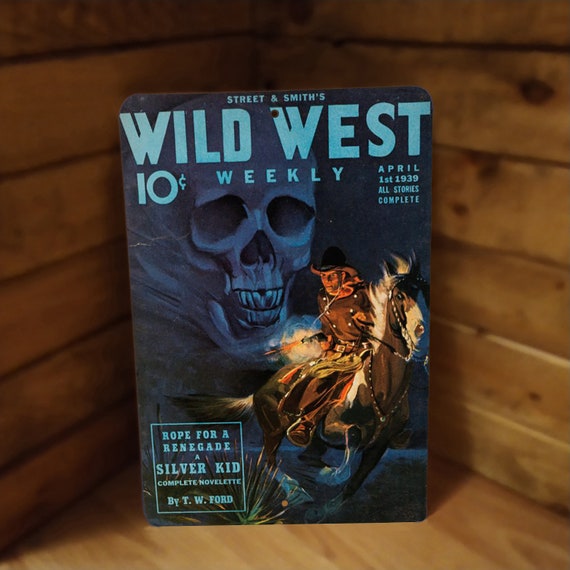In the image, a graphically rich magazine cover leans in the corner of a room where two walls with dark brown wood paneling meet, reminiscent of a log cabin. The wood features noticeable knots, particularly in the upper right corner, and the floor beneath is also made of matching dark brown boards. 

The magazine, titled "Street and Smith's Wild West," has a prominent blue header. "Wild West" is written in large block letters spanning across the top, interrupting a small hanging hole. Beneath it, the cover notes "10¢ Weekly, April 1st, 1939, All Stories Complete." In the lower left corner within a blue box, it reads, "Hope for a Renegade, A Silver Kid Complete Novelette by T.W. Ford." 

The cover artwork features a dramatic scene: a large blue skull looms in the background, while in the foreground, a man rides a galloping horse, aiming and firing a gun with smoke trailing from the barrel. The illustration appears to capture a tense moment of action, likely set at night.